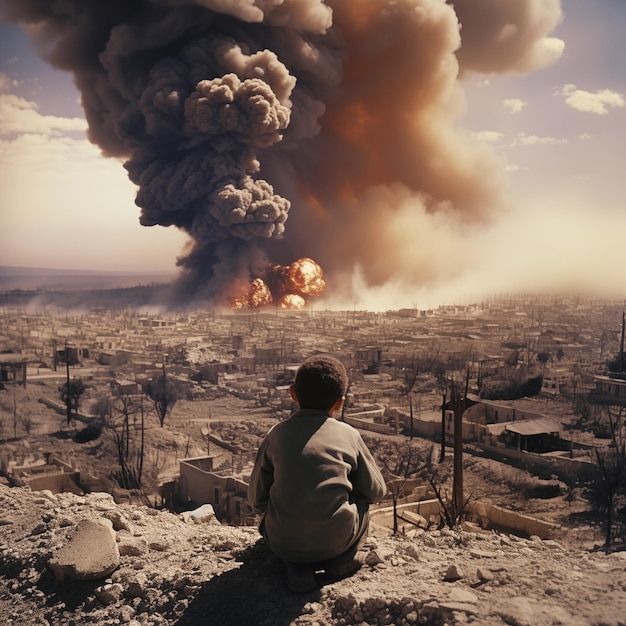In this digitally composed image, a child, possibly African American, sits on a ledge of broken rocks, gazing at a massive explosion in the distance. The child, viewed from the back, has dark brown hair and is dressed in a long-sleeved, light brown shirt, and taupe-colored pants. The scene before him is a desolate town, marked by shades of brown and featuring small, modular stone or clay houses, many of which seem destroyed. Spiky black trees punctuate the barren landscape. At the center of the town, a gigantic explosion sends forth a bright yellowish-orange fireball, enveloped by a thick, gray smoke cloud that ascends into the light blue sky, mingling with the white clouds and creating a massive dust and smoke plume. The sunlight casts an eerie glow onto the smoke, giving it a translucent appearance on the right where the orange flames shine through the thick, puffy brown clouds. The contrast between the peaceful sky and the chaotic destruction below is striking, as the child silently observes the cataclysmic scene.